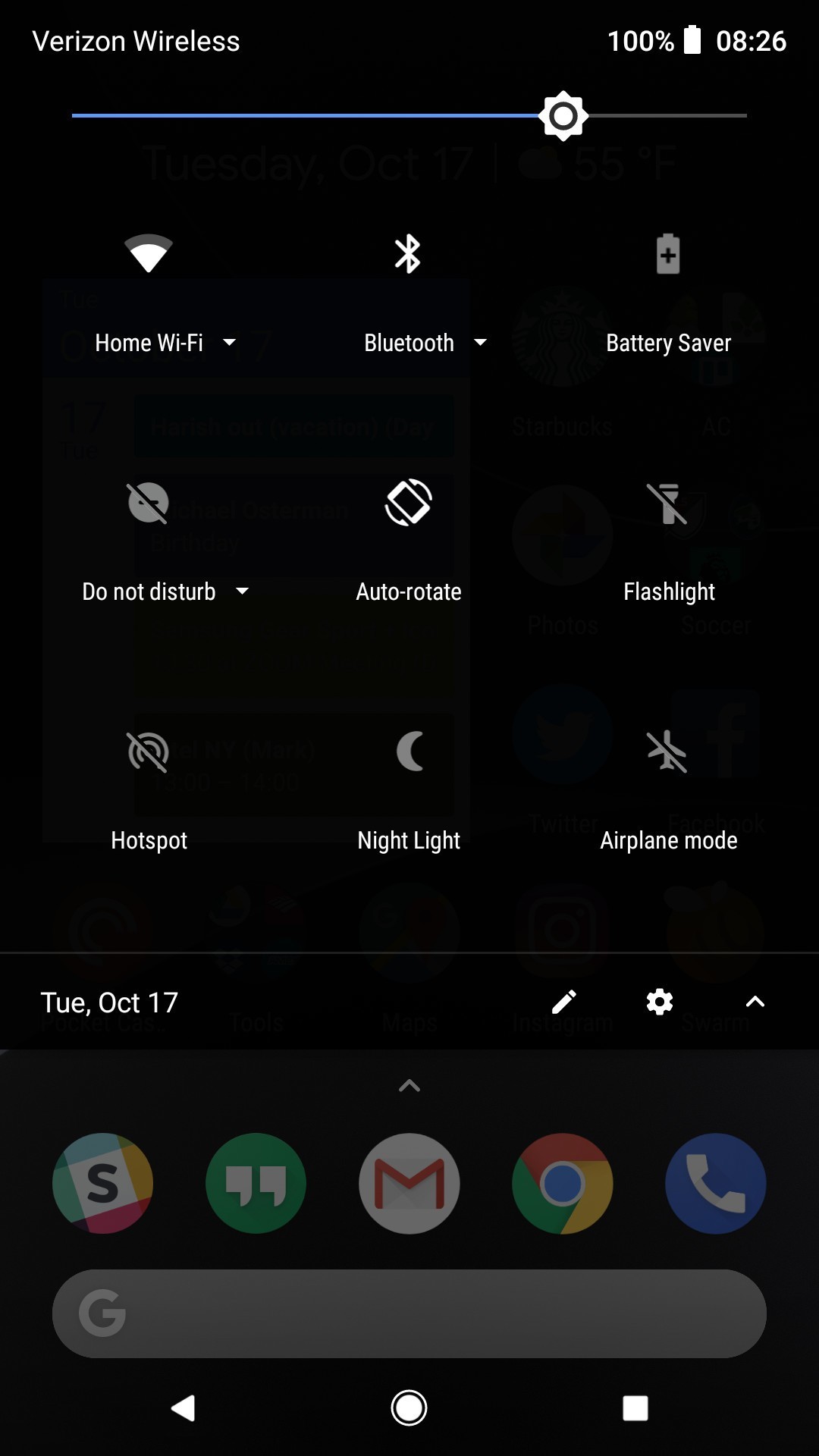This vertical image, captured on a smartphone, features a sleek, black background devoid of texture or dimension. Situated in the top-left corner, in white text, is the label "Verizon Wireless." The top-right corner displays a full battery icon at 100% and the current time, "08:26." Below this, a status bar stretches across the screen, predominantly blue with a settings icon and a gray segment.

The screenshot shows a grid of functional icons arranged across three rows. The first row includes Home Wi-Fi, Bluetooth, and Battery Saver options. The second row presents Do Not Disturb, Auto-Rotate, and Flashlight icons. In the third row are Hotspot, Night Light, and Airplane Mode. Displayed prominently in the middle of the screen is the date, "Tuesday, October 17th," accompanied by a writing icon, a settings symbol, and an upward arrow.

At the bottom, a series of circular icons line up to represent various applications: Chrome, Phone, Messaging (M), and another app marked with an "S." This section also includes the Google search bar featuring a triangle, circle, and square icon aligned from left to right, positioned at the bottom-right corner.